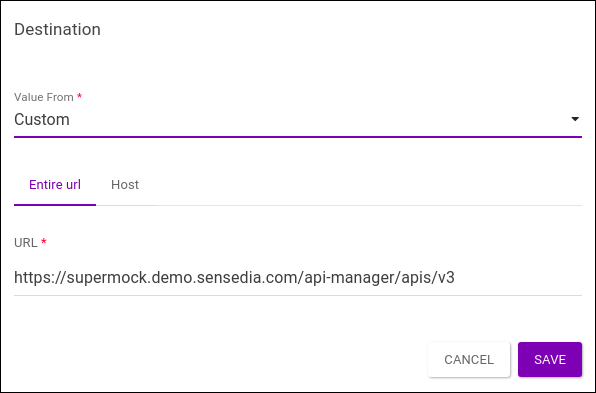The image showcases a boxed section with specific details. In the upper left corner, it prominently displays the word "Destination." Directly below this, the text "Value from custom" is shown, with the word "custom" underlined and in purple. Additionally, an entire URL is also presented in purple beneath the word "custom." The detailed URL given is "https://supermock.demo.censdia.com/.api-manager/.apis/.b3", which is marked with an asterisk. The term "Value from" is also marked with an asterisk, making these the only two asterisks visible on the page. In the lower right corner of the image, there are two buttons labeled "Cancel" and "Save."